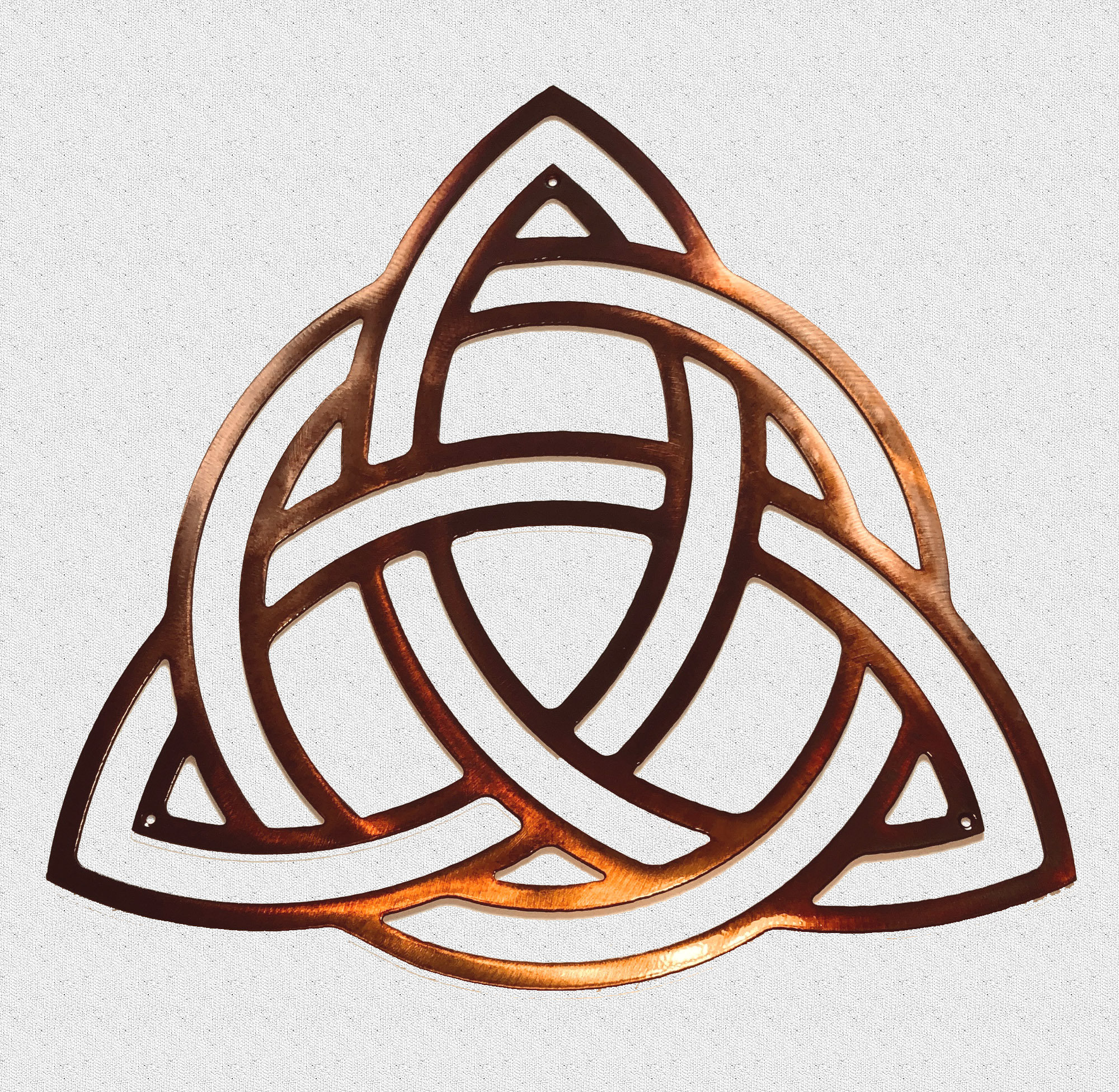The image depicts a Celtic-inspired symbol crafted from copper or bronze, showcasing a geometric, intertwined design. The symbol, primarily flat and uniformly thick, features three primary points—one at the top, one at the bottom left, and one at the bottom right. These points create a triangular shape at the core, further intricately connected by a series of intertwining curves that loop through and around each other. The central aspect of the symbol is a circle, lending an additional layer of symmetry and complexity to the design. 

It has three visible holes at the edges of the points, suggesting it is designed to be mounted onto a flat surface, likely for decorative purposes. The background of the image is plain, possibly white or gray, emphasizing the brassy or golden tones of the symbol. The metal piece resembles a crest or a three-point Celtic knot with spherical elements, hinting at its cultural significance. 

The precision of the curved, interconnected lines and the distinct brassy gleam, especially where it catches the light, accentuates the elaborate craftsmanship of this ornamental, wall-hanging sculpture.